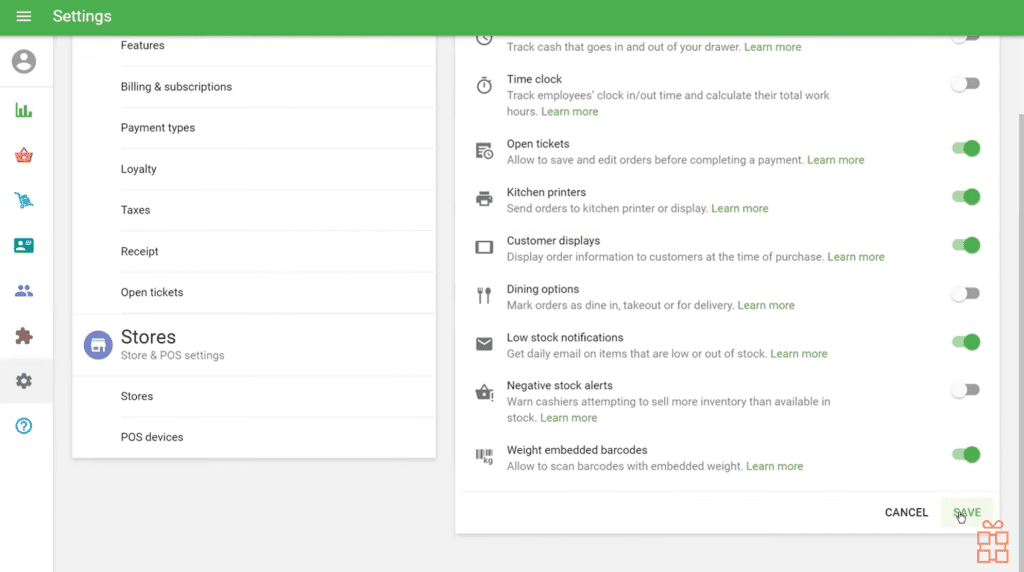Detailed Caption: 

This image showcases a settings interface from a website or an app. The top-left corner features a common menu icon represented by three white horizontal bars stacked on top of each other, situated next to the word "Settings," also displayed in white text. The background is a light green shade that spans the entire left side and extends across the top to the right side.

On the left side of the screen, a circular profile icon is prominently placed, followed by a vertical column of eight distinctive logos each representing different functions: a chart icon, a shopping cart icon, a hand holding a lightning bolt icon, a credit card icon, a two people icon, a puzzle piece icon, a gear icon, and a circle encompassing either an exclamation point or a question mark.

Adjacent to these icons, on the right, is a vertical rectangular section with a white background containing a list of options. Starting from the top, the list includes: "Features," "Billing and Subscriptions," "Payment Types," "Loyalty," "Taxes," "Receipt," and "Open Tickets." Below these options, a separate section named "Stores and POS Settings" is shown, with subsections titled "Stores" and "POS Devices."

At the bottom right corner of the image, an orange present icon accented with four small squares is displayed, adding a pop of color to the interface.